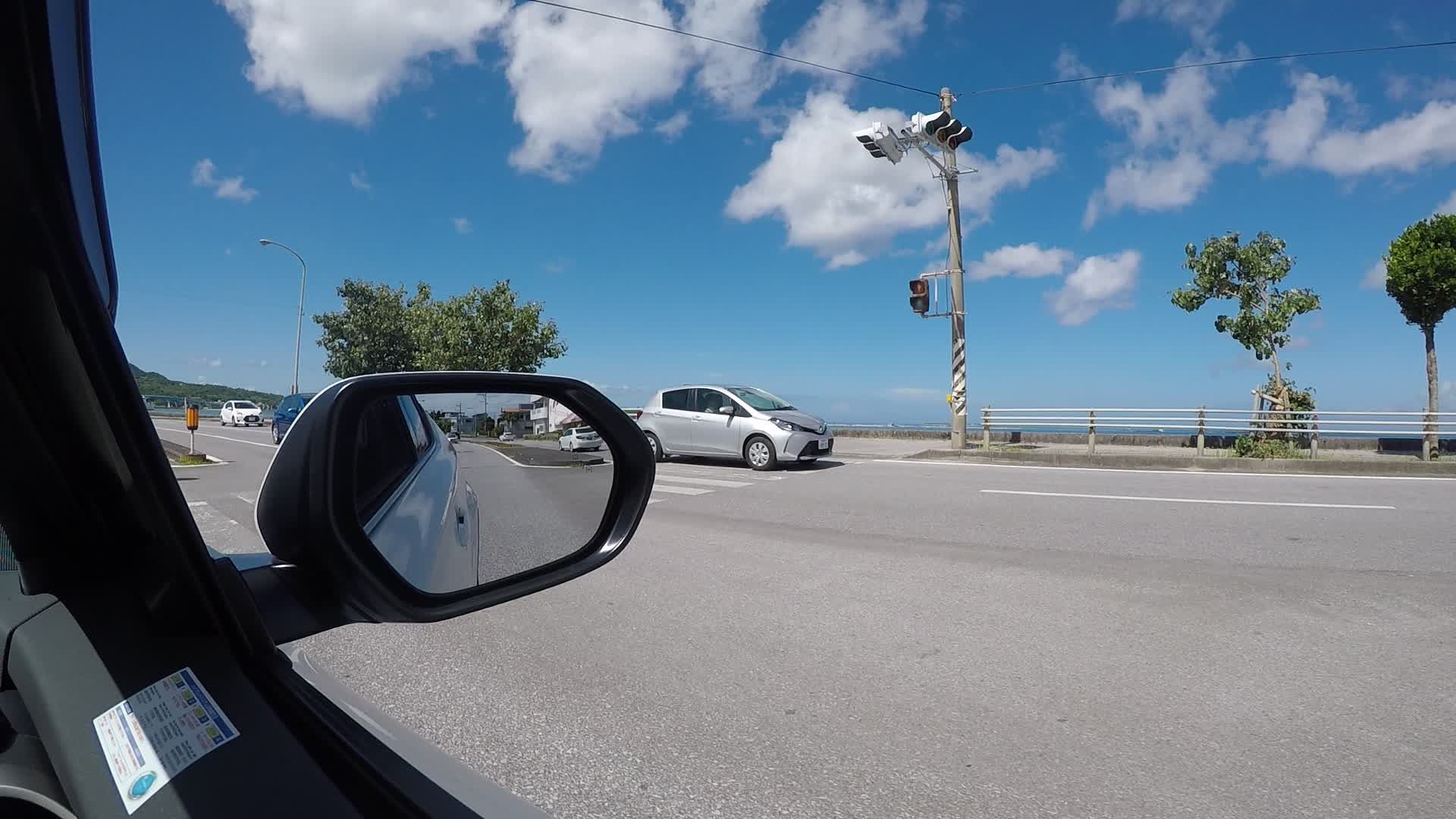This image captures the view from the front passenger side of a vehicle, taken through the window of the passenger side door. On the left side of the image, the interior curve of the vehicle's frame is visible, displaying gray metal trim. The side mirror, which is black with a reflective surface, is shown pointing rearward. The vehicle in which the photo is taken appears to be silver.

In the distance, the image reveals several lanes of traffic on a gray asphalt road. Sparse trees dot the landscape, and a bright, blue sky with a few wispy clouds suggests a clear and pleasant day. Across the lanes, a gray car is noticeable, along with glimpses of a blue car and a white car further in the background. A white railing runs along the right side of the image, though its details are indistinct. In the far distance, faint green mountains can be seen, adding a touch of natural scenery to the urban setting.